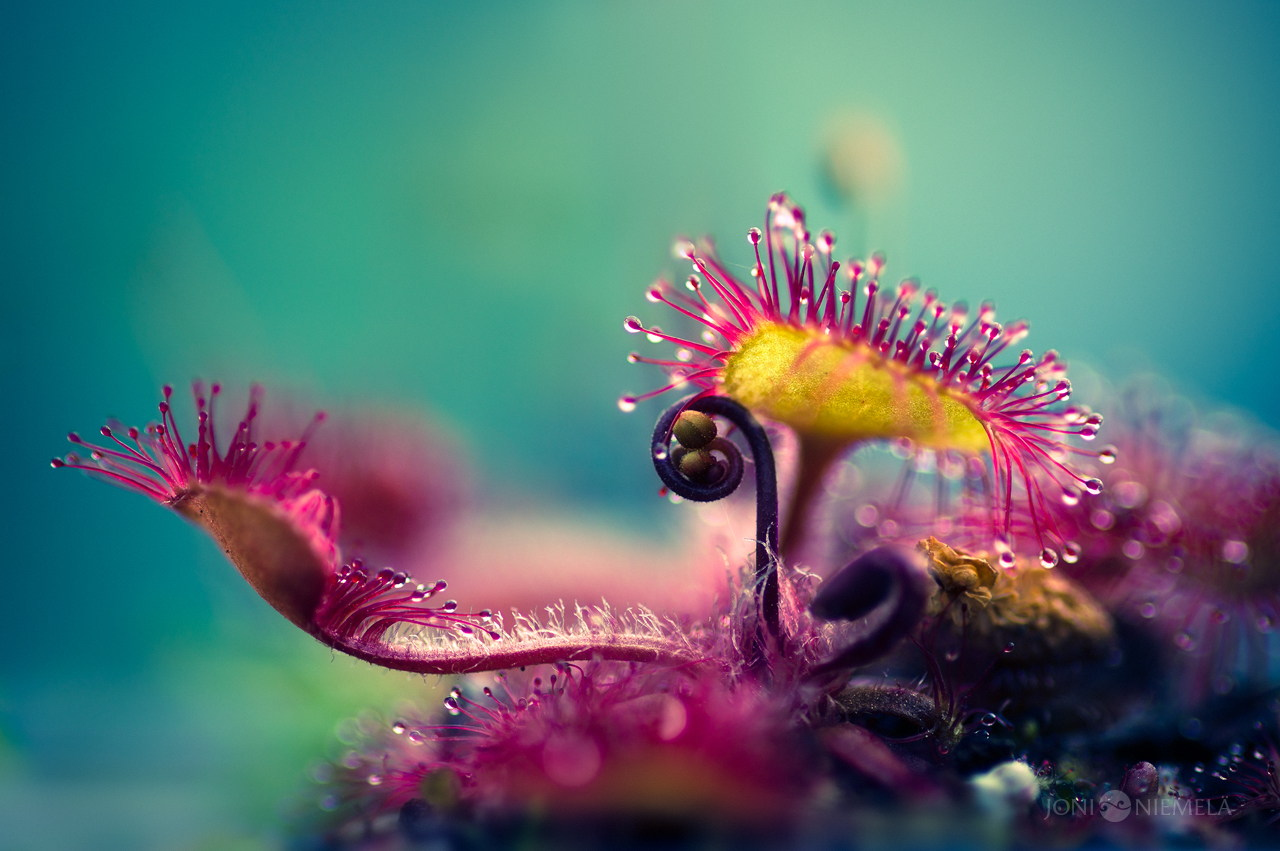In this underwater photo, an exotic aquatic plant dominates the scene with its vibrant and detailed morphology. The plant features striking purple-pink trichomes capped with droplets, lending a sense of delicate intricacy. Interspersed among these trichomes are white hairs, adding to the texture. The plant also displays areas of orange and yellow coloration, creating a vivid contrast against the predominantly green aquatic background. The stems of the plant are dark purple, and the overall bubbly design of the plant evokes a sense of otherworldly beauty. The image, a close-up shot, has a bluish-green backdrop and includes a watermark on the right indicating the name of the photographer, Joni Niemiele.